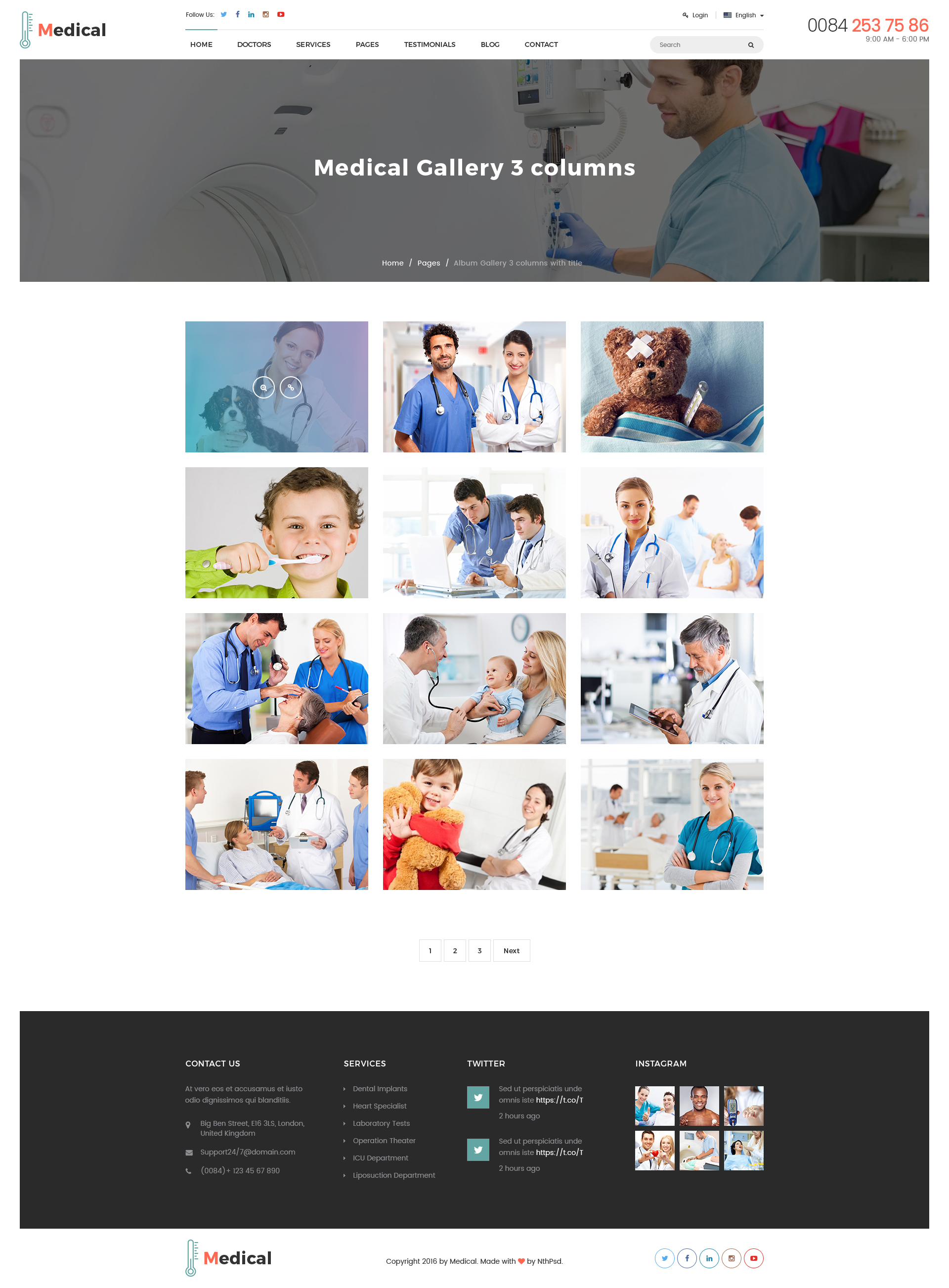The image appears to be a screenshot from the gallery section of a website. In the top-right corner, the word "Medical" is displayed, with the 'M' highlighted in orange. To the far right, a number sequence "00842537586" is visible. At the center-top, the caption "Gallery Three Columns" indicates the layout of the gallery. The gallery itself is organized into three columns and four rows of images.

In the first row:
- The first image features a doctor holding a dog.
- The second image shows two doctors together.
- The third image depicts a teddy bear with a bandage on it.

In the second row:
- The first image captures a child brushing their teeth.
- The remaining images in this row, as well as the succeeding rows, primarily feature various doctors in different settings.

Overall, the gallery displays a mix of medical professionals and health-related imagery, cohesively presented in a structured format.